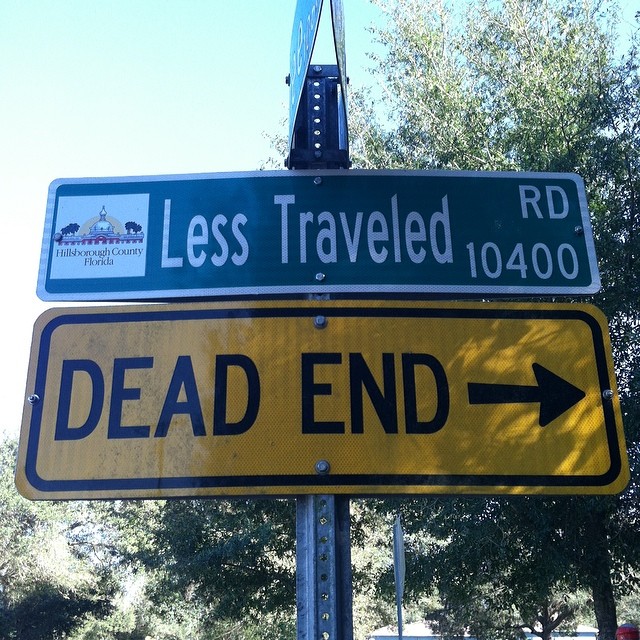This image shows a metal street sign pole with multiple signs attached to it, set against a backdrop of trees and a bright, light blue sky. The bottom sign is a large, yellow rectangular sign framed by a black line, which reads "DEAD END" in bold, capital letters, and features an arrow pointing to the right. Above this, there is a green sign with white lettering that says "LESS TRAVELED RD" and the number "10,400". The top right corner of this green sign includes the logo of Hillsborough County, Florida, depicted as a red state building with a white dome, surrounded by trees and a rising sun. The overall scene is partially shaded, with the metal pole and signs standing prominently against the contrasting bright sky. There are also two additional green street signs at the very top of the pole, angled in such a way that the text is not legible. Silver screws are visibly affixing the signs to the pole.